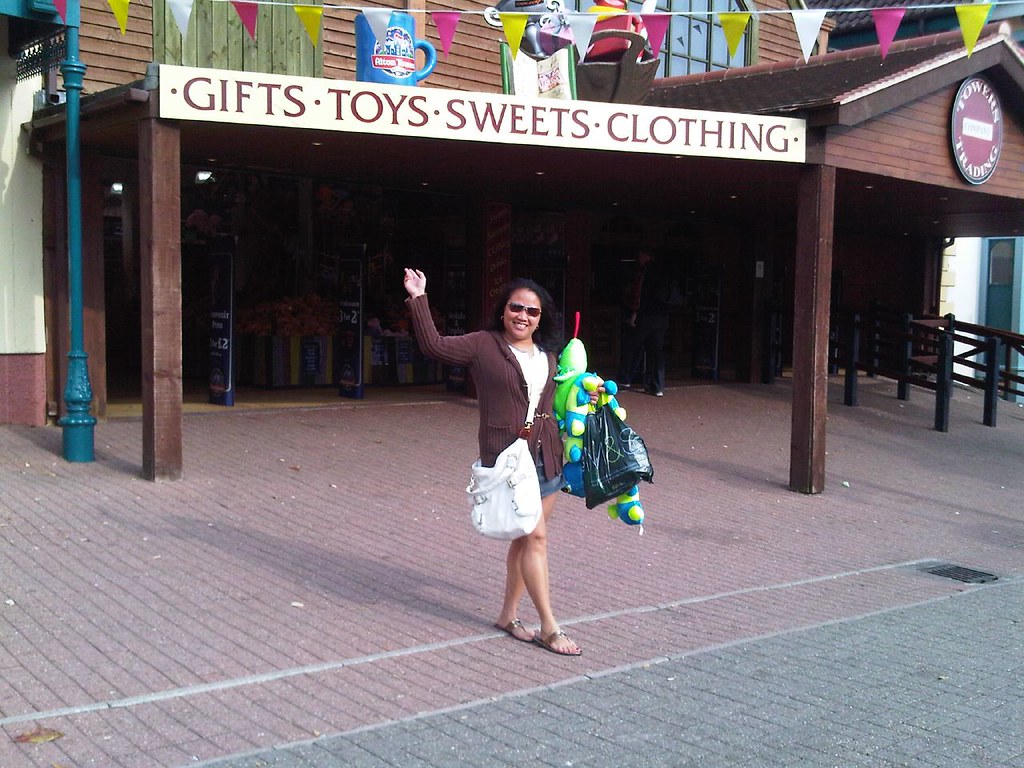A woman, dressed in a brown sweatshirt over a tan shirt and blue skirt or shorts, stands on a distinctive brick pathway - a mix of red and black bricks with white lines and a black vent. She sports sunglasses with gold trim and waves toward the camera with her right hand, while holding several stuffed animals in her left. She carries a large white bag and a smaller black bag with unreadable white text. The backdrop is a rustic log cabin-style gift shop made of brown wood, featuring brown-trimmed windows, brown wood railings, and a dark blue door with light blue trim. The shop advertises "gifts," "toys," "sweets," and "clothing" in reddish-brown letters on a sign above. Hanging above are decorative flags in red, yellow, and white strung along a white line. On the right side, there's a section of white wall bearing the text "sour trading" over a red background. A blue pole with a black gate-like feature stands on the left. The woman appears to have just exited the store, possibly a tourist attraction, looking cheerful and ready to continue her day.